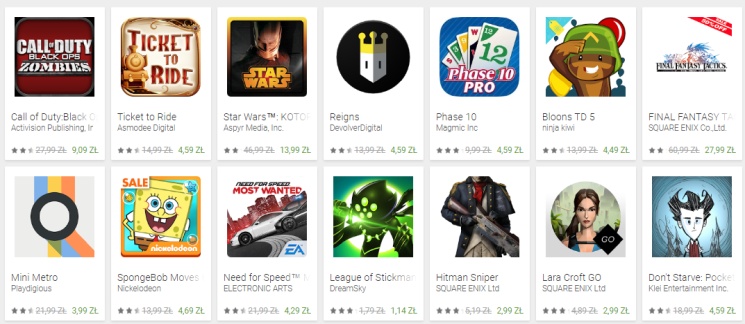The image is a rectangular interface with a gray background, displaying two rows of mini white rectangles, each containing the names and publishers of various games. 

In the first row, the games listed are as follows:
1. "Call of Duty: Black Ops Zombies" by Activision Publishing.
2. "Ticket to Ride" by ASMODEE Digital.
3. "Star Wars TM: KOTOR" by ASPYR Media Inc (partially cut off).
4. "Reigns" by Devolver Digital.
5. "Phase 10" by Magmic Inc.
6. "Bloons TD 5" by Ninja Kiwi.
7. "Final Fantasy Tactics" by Square Enix Co., Ltd.

In the second row, the titles include:
1. "Mini Metro" by PLAYDIGIOUS.
2. "SpongeBob Moves" by Nickelodeon.
3. "Need for Speed" by Electronic Arts.
4. "League of Stickmen" by Dream Sky.
5. "Hitman Sniper" by Square Enix Ltd.
6. "Lara Croft: Guardian of Light" by Square Enix Ltd.
7. "Don't Starve: Pocket Edition" by Klei Entertainment Inc.